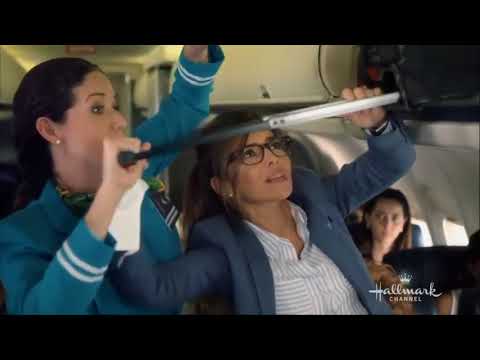This image is a detailed screenshot from a movie or television show airing on the Hallmark Channel, as indicated by the text in the bottom left corner. The scene takes place inside an airplane, where a flight attendant in a blue suit with white stripes around the wrists, identifiable by her dark black hair, is assisting a female passenger. The passenger, who has dark hair, wears black glasses and is dressed in a blue blazer with a white shirt underneath. Both women are focused on placing a black carry-on suitcase into the overhead compartment. The suitcase's handle is visible, and both appear to be struggling to fit it in properly. The passenger seems concerned, while the flight attendant helps manage the situation. Additional passengers can be seen seated behind them, with one in particular looking on from the right side of the image. A couple of airplane windows are also visible on the right, along with part of another overhead bin. All elements create a focused and detailed scenario within the confined space of an airplane cabin.